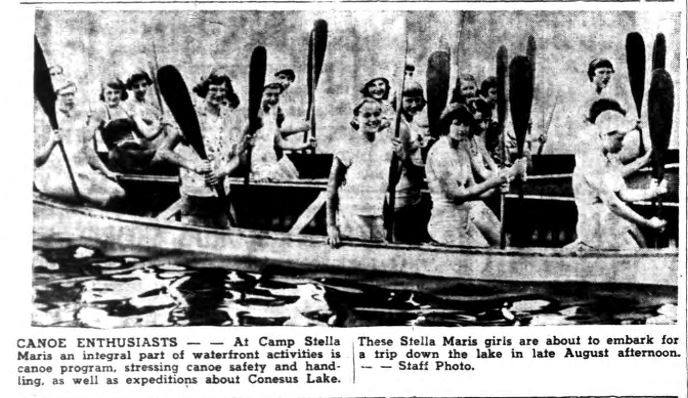This detailed black-and-white newspaper article image prominently features a photograph occupying the top three-quarters of the page, showing 15 young women sitting in two long canoes on the water. Each woman holds an upright oar, and many are smiling directly at the camera. The text beneath the image, set in black font against a light gray-white bordered, landscape-oriented layout with surrounding black lines, captions the scene with "CANOE ENTHUSIASTS" in all caps. It reads: "At Camp Stella Maris, an integral part of waterfront activities is the canoe program, which stresses canoe safety and handling, as well as expeditions around Canesis Lake. These Stella Maris girls are about to embark on a trip down the lake on a late August afternoon. Staff photo." The style evokes a vintage newspaper print ad.